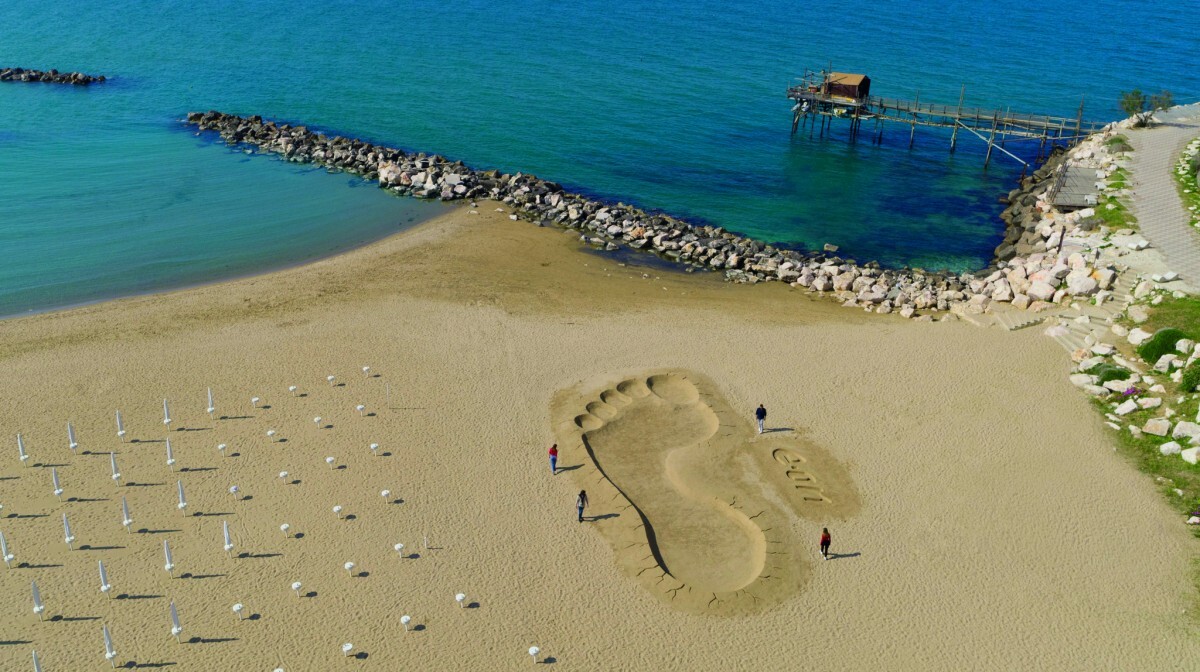The image depicts a picturesque beach scene with meticulously arranged white chairs and umbrellas, creating a sense of order and tranquility. At the center of the beach, a massive imprint of a foot is prominently visible in the sand, with an inscription that intriguingly appears to resemble the word "gun," though it's likely a different word. Surrounding the imprint, groups of people stand curiously, adding liveliness to the scene.

To one side of the beach, a collection of white rocks is crumbled and scattered, extending out into the ocean. Beyond these rocks, the beach continues, offering a similar stretch of sandy shoreline. This rock formation creates a natural jetty, providing a calm, sheltered swimming area with minimal waves, ideal for a serene dip in the water.

On the opposite side of the rocks, a charming pier extends into the water, leading to a quaint little house at its end. This house, resembling a chateau, adds a touch of architectural elegance to the coastal landscape. The entire setting exudes a blend of natural beauty and subtle human touches, inviting viewers to imagine a peaceful day at this idyllic seaside retreat.